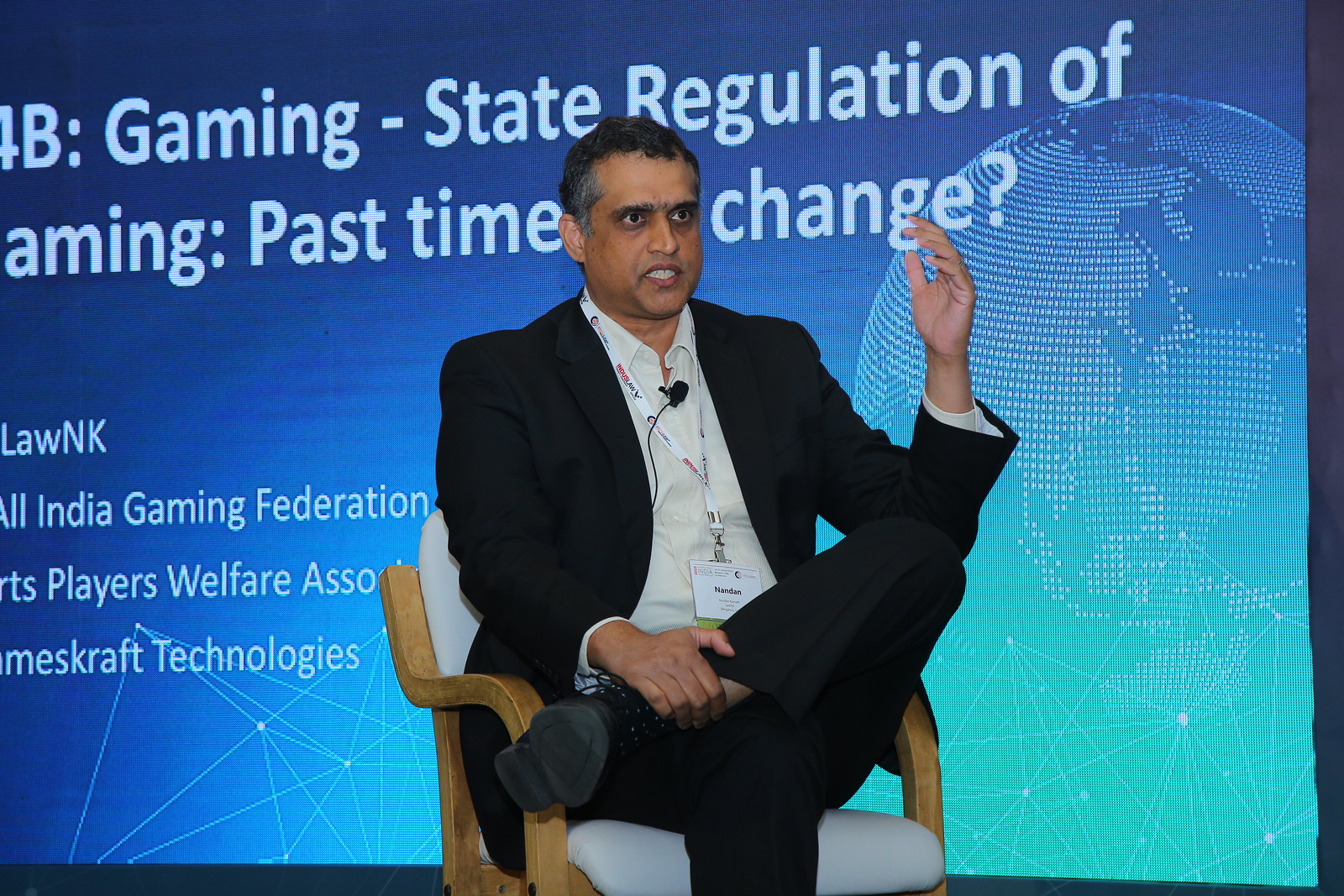The image depicts a man seated in a white-cushioned chair with wooden armrests, looking directly at the camera. He is dressed in a black suit, beige collared shirt, and black shoes. A lanyard with a name tag hangs around his neck, and a small black microphone is clipped to his shirt. The man has short, dark hair with salt-and-pepper graying at the temples, and he's of Indian descent with a brown skin tone. Behind him is a large LED screen displaying the title "4B Gaming: State Regulation of Gaming, Past Time for Change?" in white lettering against a blue background. Additional text on the left side of the screen is partially obscured but mentions the "All Indian Gaming Federation Players Welfare Association" and "Games Craft Technologies." The screen also features a globe composed of white dots with a wireframe design on the right side. The man appears to be engaged in a discussion or presentation about gaming regulations, exuding a focused and determined demeanor.